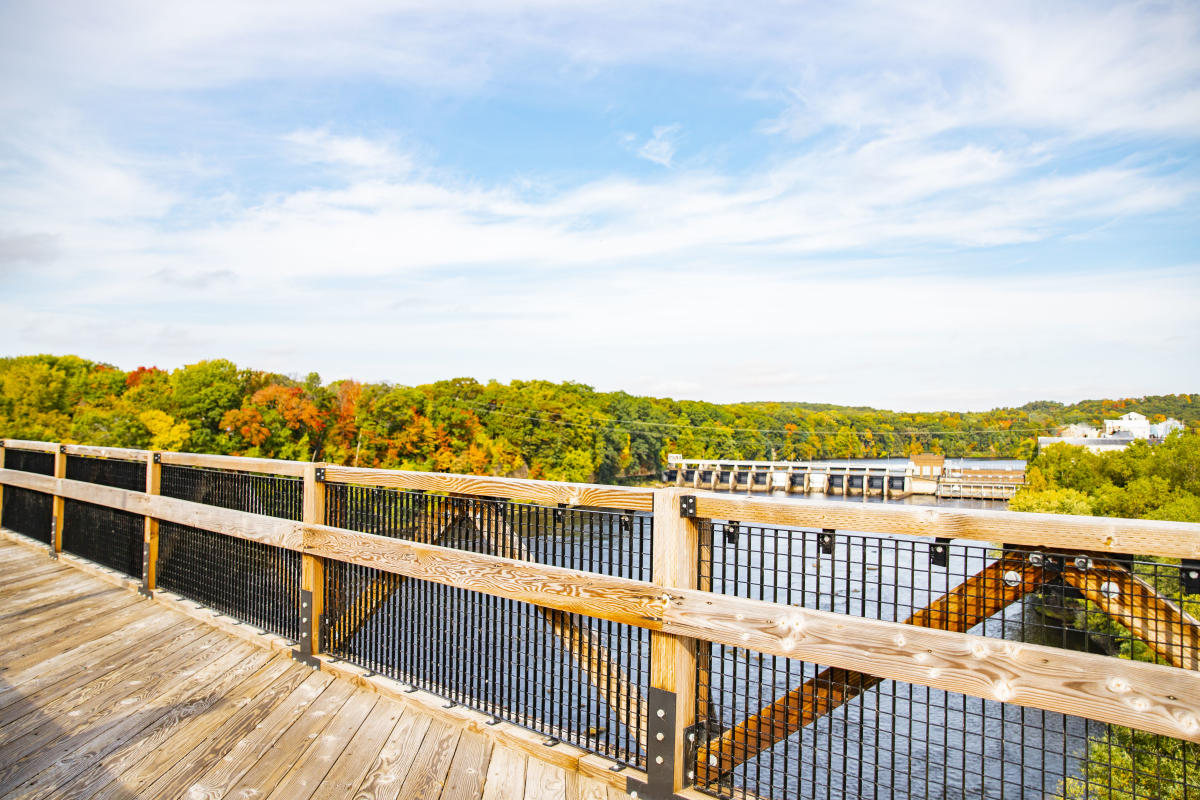An outside landscape photograph captures a serene scene with a light blue sky adorned with whispery white clouds. The image prominently features a wooden bridge with sturdy planks and wooden railings, intertwined with black metal mesh to ensure safety. The bridge stretches over a calm river. On both sides of the river, dense, lush green trees dominate the landscape, interspersed with patches of fall foliage, showcasing leaves turning vibrant shades of red, yellow, and orange. In the distance, another bridge, covered and structured differently, peeks through the heavily treed backdrop. The main focus remains on the wooden bridge in the foreground, accentuating its rustic charm against the contrasting natural elements.